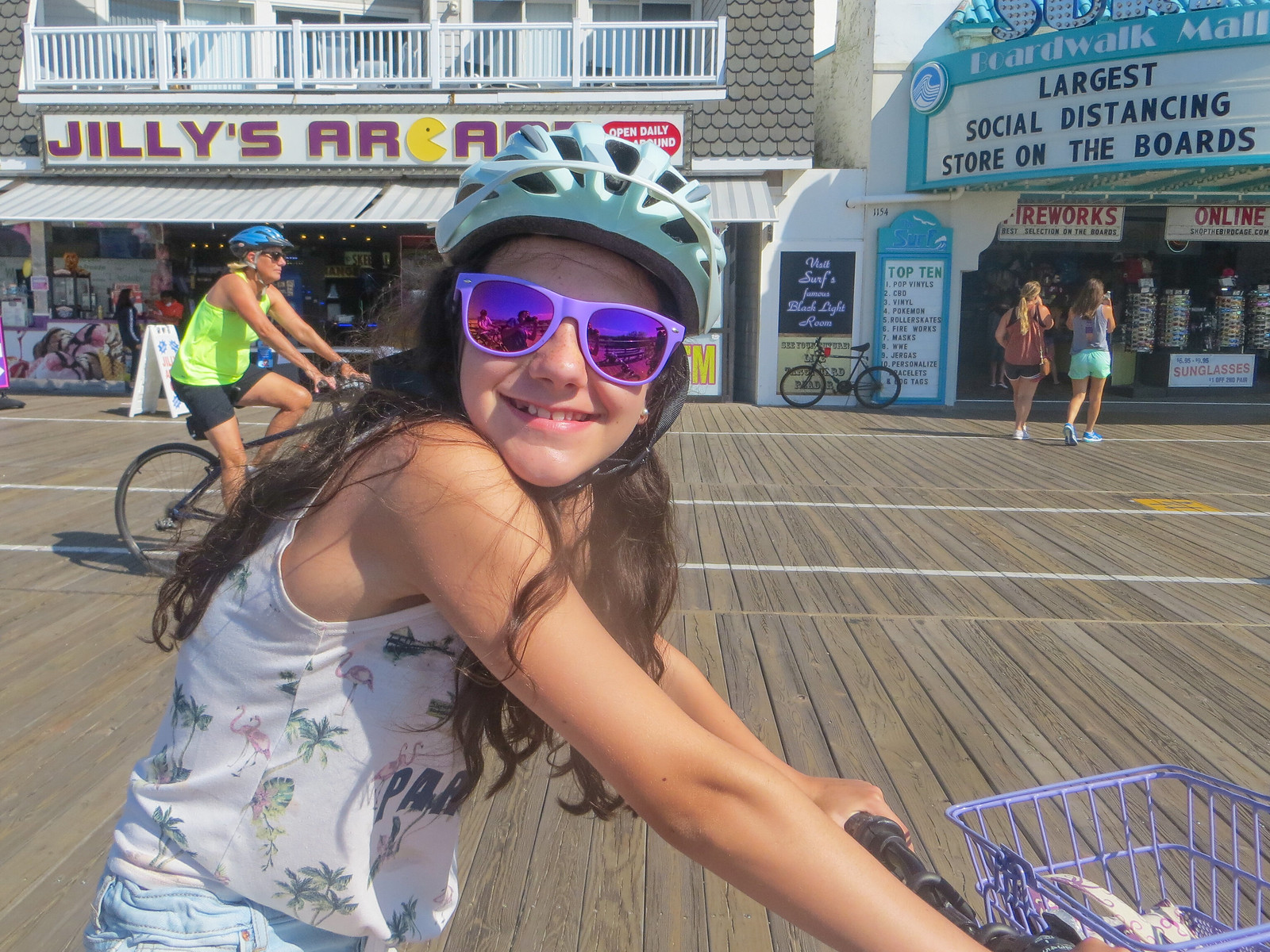The image captures a lively outdoor scene dominated by a young girl joyfully riding a bicycle adorned with a purple basket. She sports vibrant purple sunglasses, a light blue bike helmet, and a sleeveless white tank top decorated with flamingos. The wooden plank boardwalk stretches behind her, populated by people enjoying the day. A woman in a bright green sleeveless top, black shorts, and a blue helmet rides another bike nearby. Further back, two women in summer attire stroll leisurely.

Visible shop fronts add context to the scene, with signs advertising local attractions and sales. A prominent sign for "Jilly's Arcade" declares it open daily, while another for the "Boardwalk Mall" touts it as the largest social distancing store on the boards, listing a variety of items such as fireworks and top ten pop vinyls. Other advertisements highlight specials, like sunglasses priced between $6.95 and $9.95 with a discount on the second pair, and enticing invitations to visit Surf’s famous black light room. The scene is a vibrant slice of boardwalk life, filled with summer activity and commercial buzz.